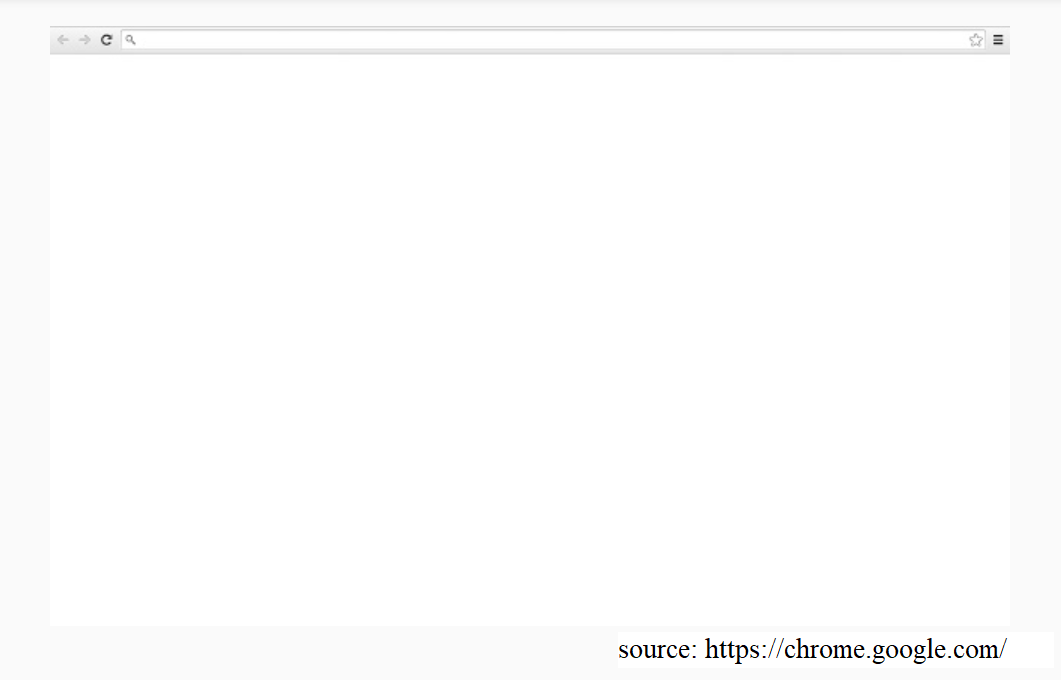This screenshot captures an empty Chrome browser window displaying a blank white page. The URL bar at the top is entirely empty, containing no web address or search query. On the left side of the toolbar, there is a magnifying glass icon followed by back and forward navigation buttons, and a refresh page icon. On the far right side of the toolbar, a star (likely for bookmarking) and a three-bar menu icon (indicative of Chrome’s settings menu) are visible. At the bottom right corner of the screen, the text "source" is displayed alongside the URL "https://chrome.google.com".